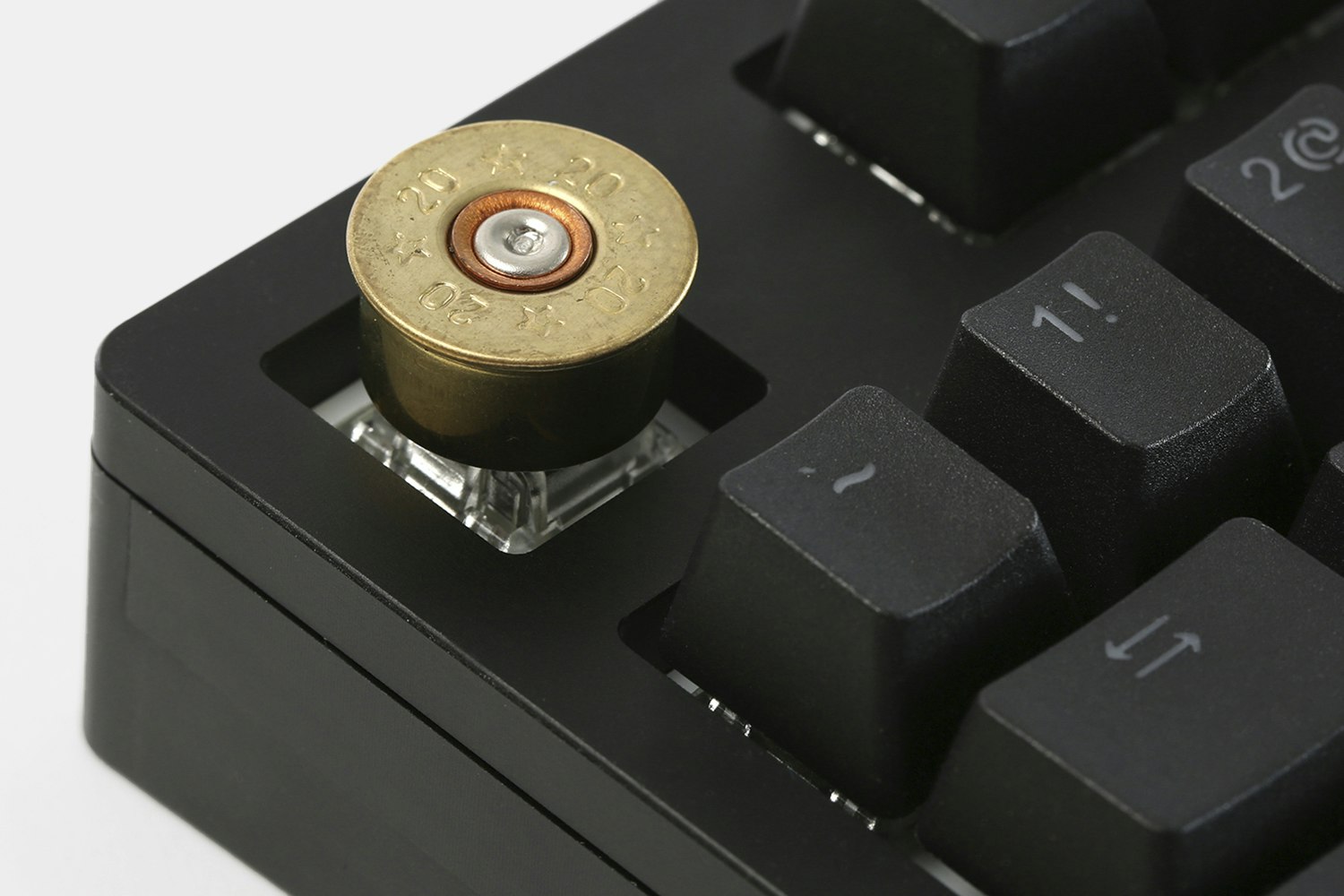The image showcases an extreme close-up of the upper left corner of a black keyboard, focusing on the Escape (Esc) key. The usual Esc key cap has been uniquely replaced with the back end of a revolver bullet shell. This custom key cap features the metallic, circular end of a bullet, with a gold-colored top engraved with the number "20" and several small stars repeating around its circumference. The inner circle of the bullet’s casing is copper or metallic in color, highlighted by a brass ring around it, giving it a distinctive, eye-catching appearance. The keyboard's switches are clear, and the background of the image is white, enhancing the contrast and emphasizing the unique key cap.